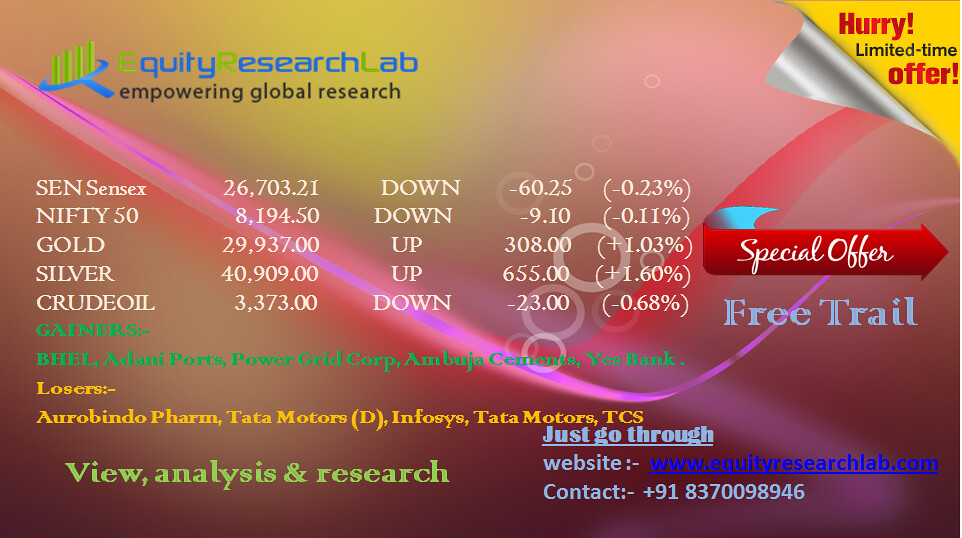This image features an advertisement from Equity Research Lab, showcasing stock and commodity data. The background is yellow with pink swirls, giving a vibrant look. In the top right, there's a striking curl-over effect, making it appear as if the page corner is lifted, revealing the message "Hurry, limited time offer!" in red and black text on a yellow backdrop. The top left corner proudly displays the logo and name "Equity Research Lab" in green and blue lettering, followed by the tagline "Empowering Global Research" in black.

The center of the image contains vital stock stats, listing the names of resources such as Sensensics, Nifty Fifty, Gold, Silver, and Crude Oil, along with their recent prices and percentage changes. The information is organized in two sections: "Gainers" in green and "Losers" in yellow, each listing various corporations.

The bottom of the advertisement features two call-to-action messages. On the left side in green text, it says "View Analysis and Research," while the right side in blue text reads "Just Go Through" followed by "Website: equityresearchlab.com" in a blue hyperlink style and the contact phone number including the country code +91.